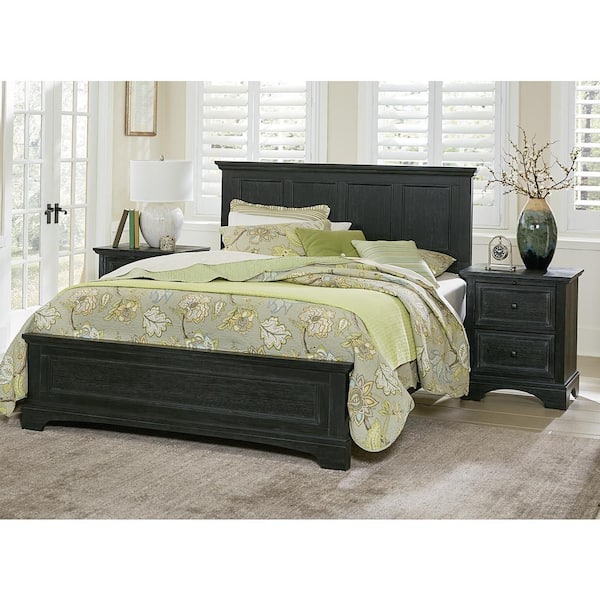This is a detailed photographic image of an indoor bedroom scene, with its most prominent feature being a centrally positioned bed. The bed boasts a high, dark brown headboard and matching footboard, with a bedding ensemble that includes a light green, dark green, and beige floral print comforter and pillows. The pillows' colors include light and dark green, as well as beige, enhancing the floral theme. The white linen sheet and the blanket with the floral print add a touch of softness.

Flanking the bed are two wooden side tables, each with two drawers. On the right side table, there's a green vase containing plants, possibly pussy willows, alongside an arched, old-fashioned clock. The left side table supports a white lampshade, and next to it, a few books lean against the wide lamp base. Behind the headboard is a set of white-framed Venetian blind-style windows, flooding the room with natural light.

To the left of the bed, a pair of double glass doors with dark knobs offer an additional point of interest. The floor features a gray carpet that complements the light tan walls, creating a warm and inviting atmosphere. In the upper left corner of the photo, a framed picture is visible, though the details within it are unclear.

The overall arrangement and color palette, combined with the floral prints and wooden elements, create a cohesive and tranquil bedroom setting.